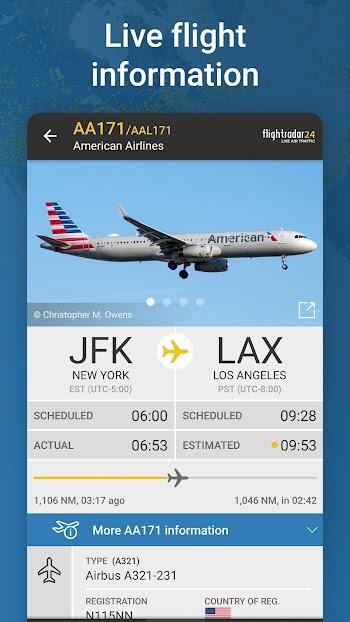This screenshot, likely from a website, showcases live flight information with a high-contrast light blue and dark blue duotone background, possibly a pattern or photo. The focal point appears to be an outline of a smartphone screen displaying the flight details, exemplifying how one can view flight information on their device. 

At the top of the screen, there is a gray bar that reads "AA-171 / AAL-171," indicating an American Airlines flight, with the information sourced from Flight Trader 24, a live air traffic tracking application. Below this, a photograph portrays an American Airlines airplane in flight, with four different photo options available.

The flight in question is from JFK (New York) to LAX (Los Angeles). A yellow plane icon on the display marks the flight's current position between the departure and arrival airports. The time zones for each airport are indicated, with JFK listed as UTC-5 and LAX as PST (UTC-8). The scheduled departure time is 6:00, however, the actual departure time is 6:53. The scheduled arrival time at LAX is 9:28, with an estimated arrival now at 9:53.

A visual representation of the flight's progress shows a plane moving from left to right, with a yellow bar indicating the completed portion and a gray bar showing the remaining distance. The flight has covered 1,106 nautical miles (NM) as of 3 hours and 17 minutes ago, with 1,046 NM remaining, expected to be covered in 2 hours and 42 minutes. The entire flight duration is inferred to be approximately 5 hours.

Additional details include the aircraft type, an Airbus A321-231, with the registration number and country of registration noted as the United States. The description concludes with a prompt to read more about the flight details.